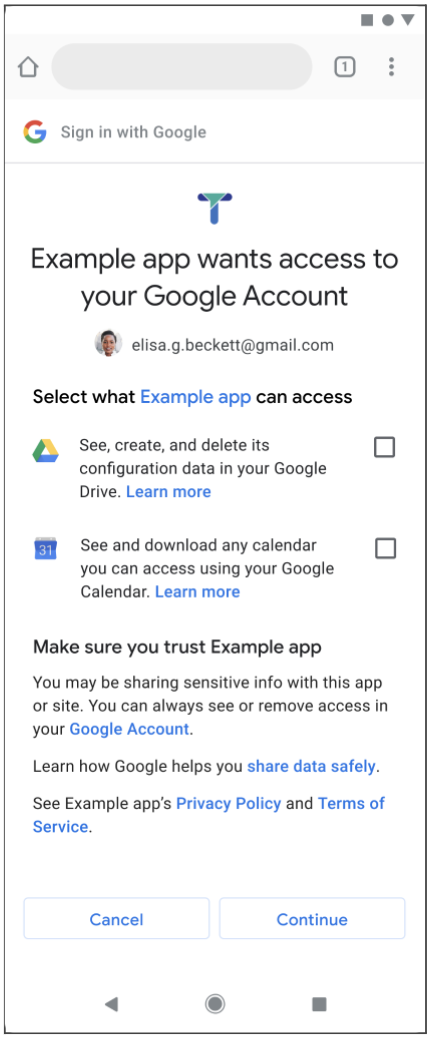Here is a detailed and cleaned-up caption based on the given description:

---

A detailed screenshot from a Google login page. Starting at the top, there is a home icon followed by a search bar, indicating that only one tab is open. To the right of the search bar, there are three vertical dots representing the menu options. Below this, the page features the Google 'G' icon and a button prompting users to "Sign in with Google." A thin gray line marks a separator, beneath which a teal and blue 'T' logo appears.

In bold black letters, the text reads: "Example App wants access to your Google Account." Next to a small circular profile picture of a light-skinned Black woman with short hair, the email address "alisa.g.beckett@gmail.com" is displayed.

Further down, in black text, it says "Select what" followed by "Example App" in blue text and then "can access" in black text. Below this, there are permissions listed:

1. A Google Drive icon in green, blue, and yellow, with the text: "See, create, and delete its configuration data in your Google Drive." Following this, "Learn more" is clickable in blue text with a checkbox beside it.
2. A Calendar icon followed by: "See and download any calendar you can access using your Google Calendar." The text "Learn more" is again clickable in blue with a checkbox next to it.

At the bottom, a cautionary message states: "Make sure you trust Example App. You may be sharing sensitive info with this app or site. You can always see or remove access in your Google Account."

---